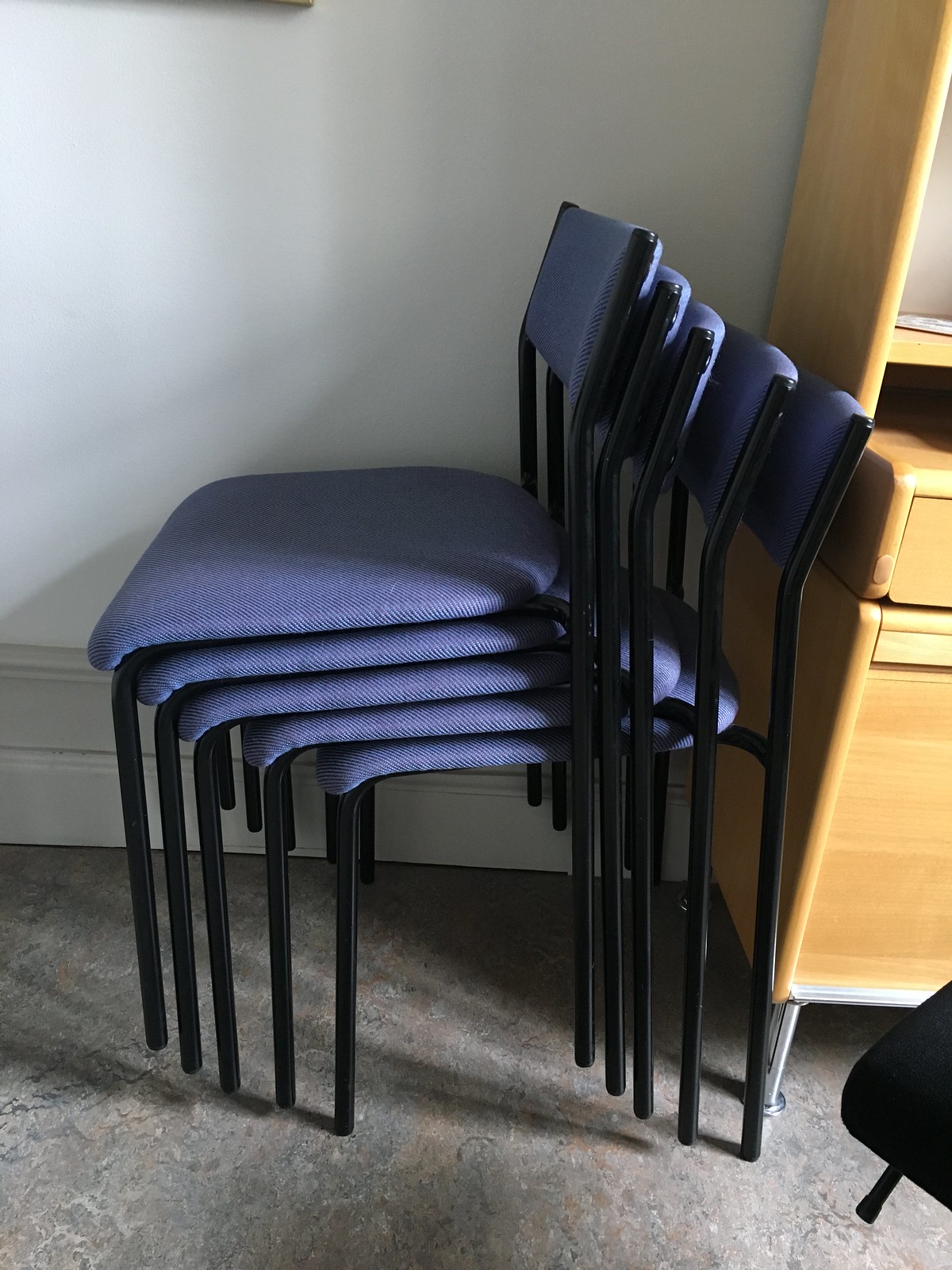The image captures a room with an unfinished grey concrete or brownish-grey linoleum floor and an off-white wall adorned with white baseboard trim. In the center of the frame, five identical blue chairs are stacked one on top of the other. Each chair features a deep royal blue cushion on both the seat and backrest, supported by a black metallic frame. The chairs appear to be toppling forward slightly. To the right of the chairs stands a light-colored wooden piece of furniture, possibly a desk or bookshelf, with a top shelf and drawers below. The legs of this furniture have a metallic finish. Also visible on the bottom right of the image is a black triangular object protruding onto the floor. The chairs, dominant in the scene, are positioned with their backs against the piece of furniture, adding a sense of precariousness to their arrangement.